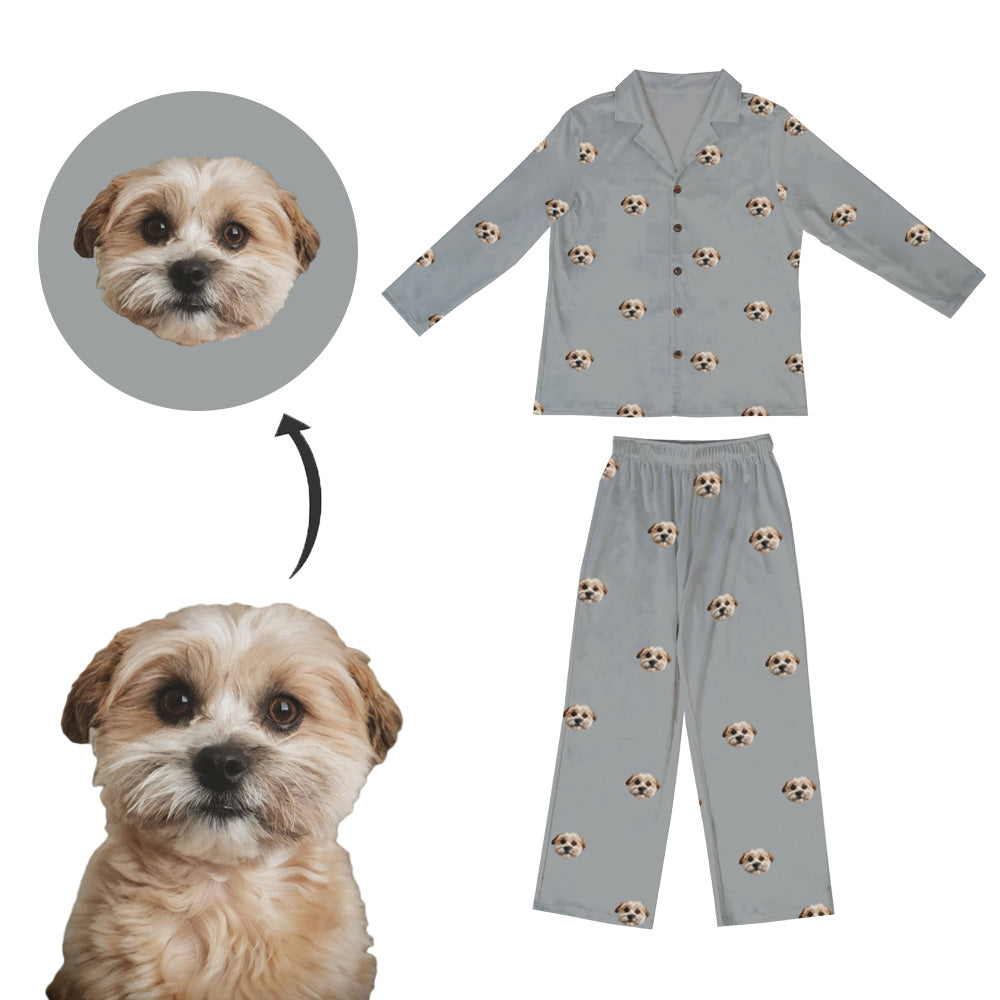This image appears to be an advertisement for customizable pajamas. The set of pajamas featured are gray with an all-over repeating pattern of a cute little brown puppy's face. The pajamas consist of long pants with an elastic waistband and a long-sleeve, V-neck top with a collar and black buttons down the front. The sides of the advertisement illustrate how you can customize your own pajamas: on the lower left is a photograph of the adorable puppy with black pupils, and an arrow points to the top left where a circular pattern featuring just the puppy's face is shown. This exact pattern is replicated on both the pajama top and bottoms, approximately 20 times per piece. The entire layout is presented on a white background for clarity, emphasizing the various stages of customization from the original puppy image to the final patterned pajamas. The result is a charming and personalized set of loungewear showcasing the beloved canine's face.